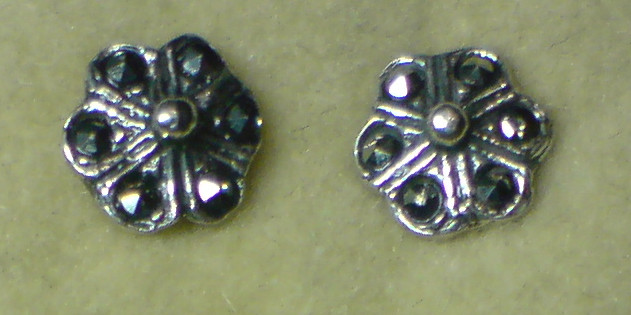The photo features a close-up of two antique-style silver earrings, each designed in a six-petaled floral motif. The earrings are meticulously crafted, with each petal adorned by a small stud or stone that protrudes through holes in the petals, adding a touch of delicate intricacy to the design. The central part of each earring features a solid round spoke, around which the floral design is structured. Between the petals, two striped grooves enhance the detailed craftsmanship. The earrings are shiny, evoking an antique aesthetic, and are silver in color. Notably, each petal's stone appears to be a dark bluish-green, adding a splash of color to the otherwise metallic piece. The earrings are placed on a green-colored table, which serves as a subtle backdrop, highlighting their intricate details.